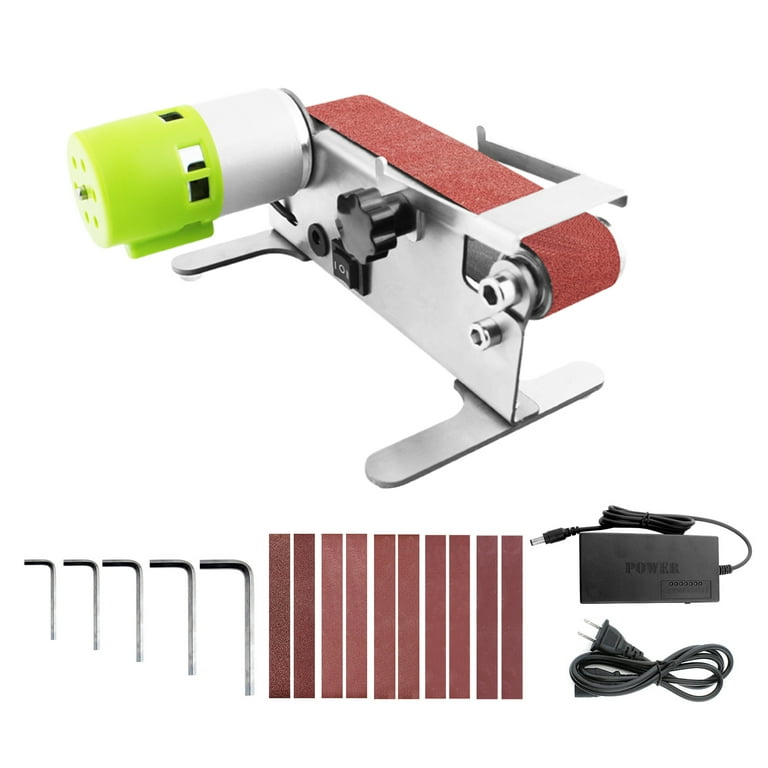This is a detailed product image of a metal sanding belt machine against a plain white background, resembling listings typically seen on home improvement websites like Lowe's or Home Depot. The main body of the machine features a rust brick red sanding belt running along the top and is constructed from a silver steel material. On the left-hand side of the belt, there is a neon orange 2-inch cylinder cap covering a metal cylinder. Adjacent to this are black control elements including a black turning lever, a black on and off switch, and a black port for plugging in the unit. 

The machine is stabilized by metal stands on either end. Below the machine in the image, accessories are neatly displayed. These include five different-sized Allen wrenches, ten sanding belts of varying grits, a black power strip, and a black power cord. Each of these components is essential for the operation and versatility of the sanding machine, ensuring it meets various sanding needs.